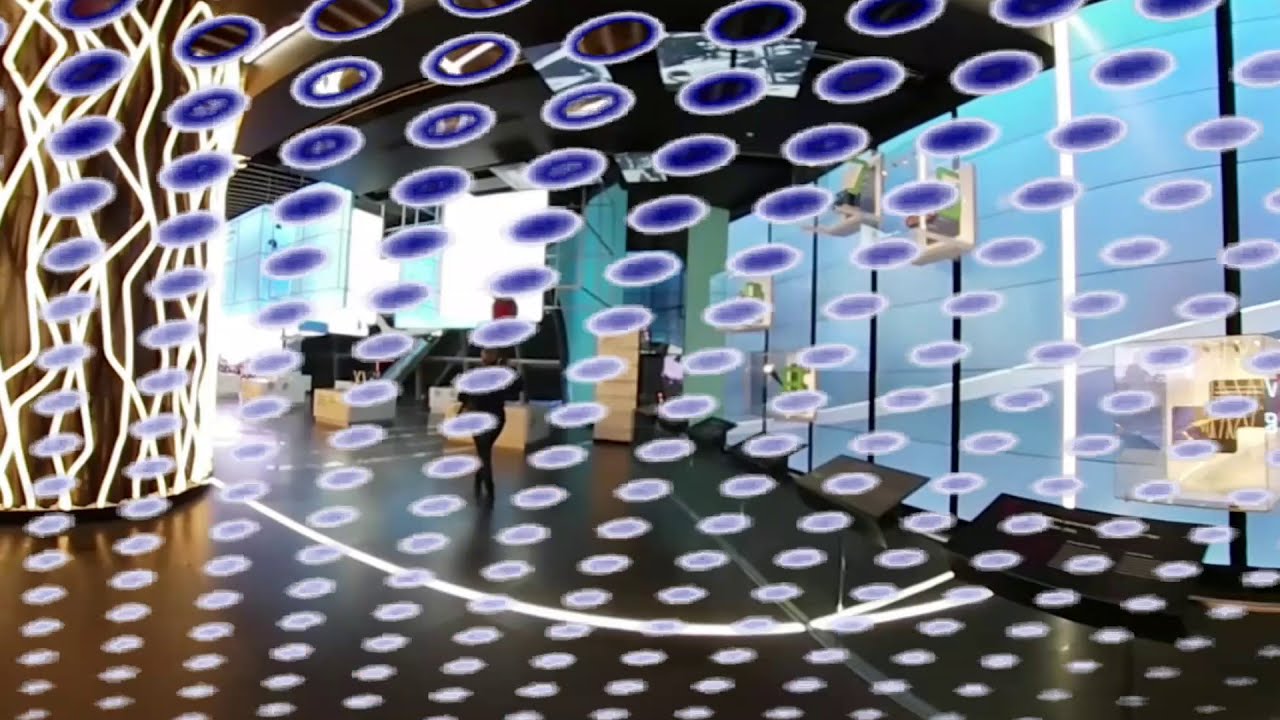The image captures the interior of a large, museum-like room with a dark, hard floor and an overall immersive atmosphere. The right side of the room features a sweeping, curved wall composed of blue, glass-looking panels that give off an impression of vastness and modernity. In the distance on the left, bright white panels of indeterminate nature add a stark contrast to the blue tones. Dominating the foreground, a mosaic of blue, oval-shaped dots with white perimeters forms a cascading, oblique pattern from right to left, resembling floating bubbles that gradually become smaller near the bottom and larger at the top.

Further details reveal a significant video screen wall adorned with stacked television screens projecting various images. Below, you can see several black signs mounted on metal posts scattered throughout the room. Additionally, a large cylindrical structure with illuminated, zigzagging LED tubes ascends from the floor to the ceiling, contributing to the high-tech ambiance. The photograph appears to be taken from behind a glass window covered in the same dotted pattern, which subtly distorts and animates the view of this visually captivating space. A single person is seen walking down the hall, subtly emphasizing the scale and dynamic essence of the environment.